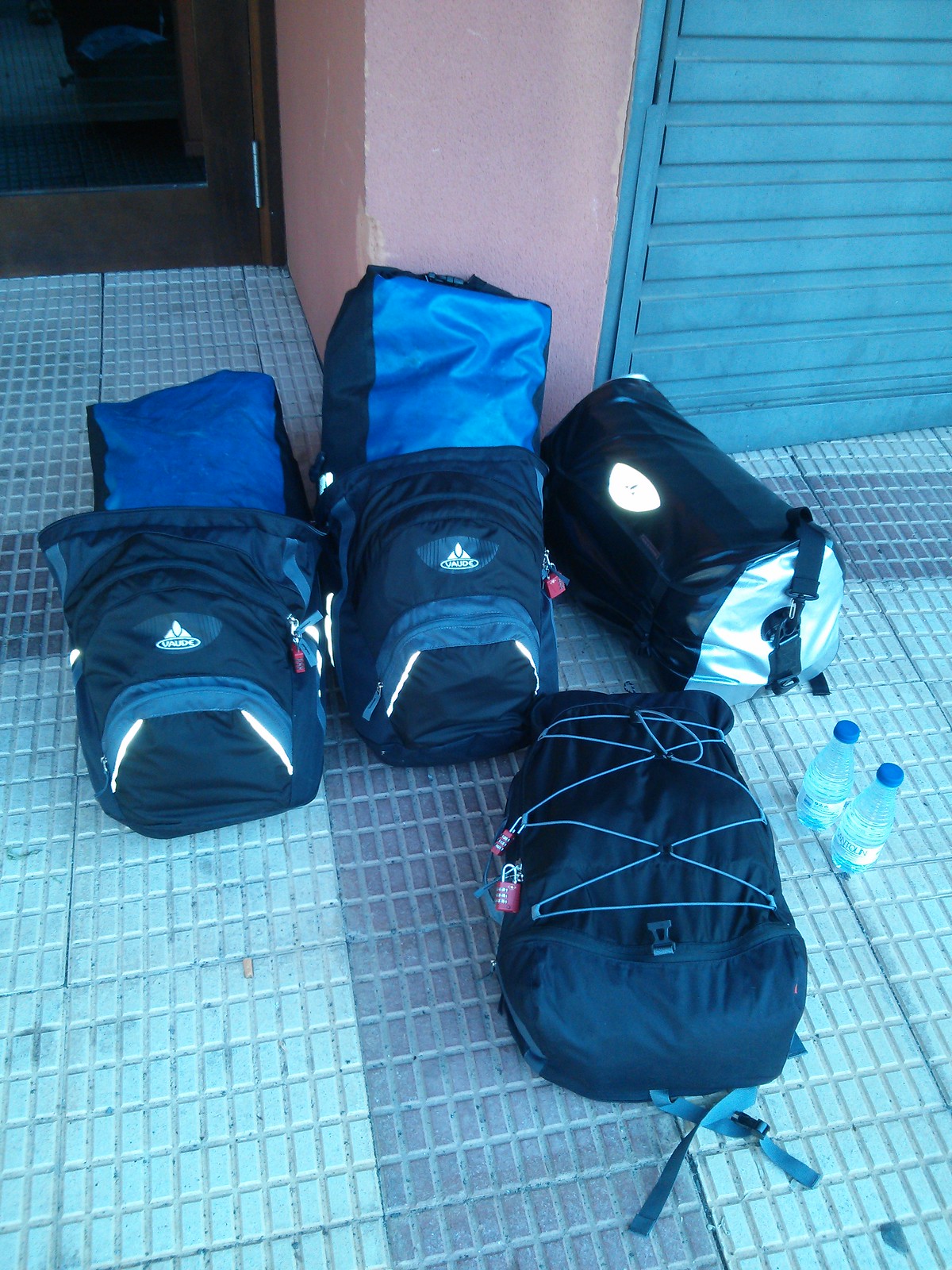This detailed color photograph captures four packed bags on a tile floor characterized by very small, rectangular, light blue tiles with darker blue stripes forming both vertical and horizontal patterns. The scene is set against a muted backdrop with a dusty pink wall featuring a turquoise panel in the upper right corner, likely a door with slats, next to the intersection of the wall and a doorframe.

Of the four bags, three rest against the wall in a back row while one lies separately in the foreground. The two identical bags on the left and center of the back row are predominantly dark blue with lighter blue rectangular logos accented with white stripes, resembling backpacks. On the right in the back row, a cylindrical-shaped duffel bag displays a silver bottom and features a logo on its side. In front and slightly to the left of this arrangement is a slate blue bag with criss-crossing light blue cords. Additionally, there are two plastic bottles with blue caps placed to the right of this final bag.